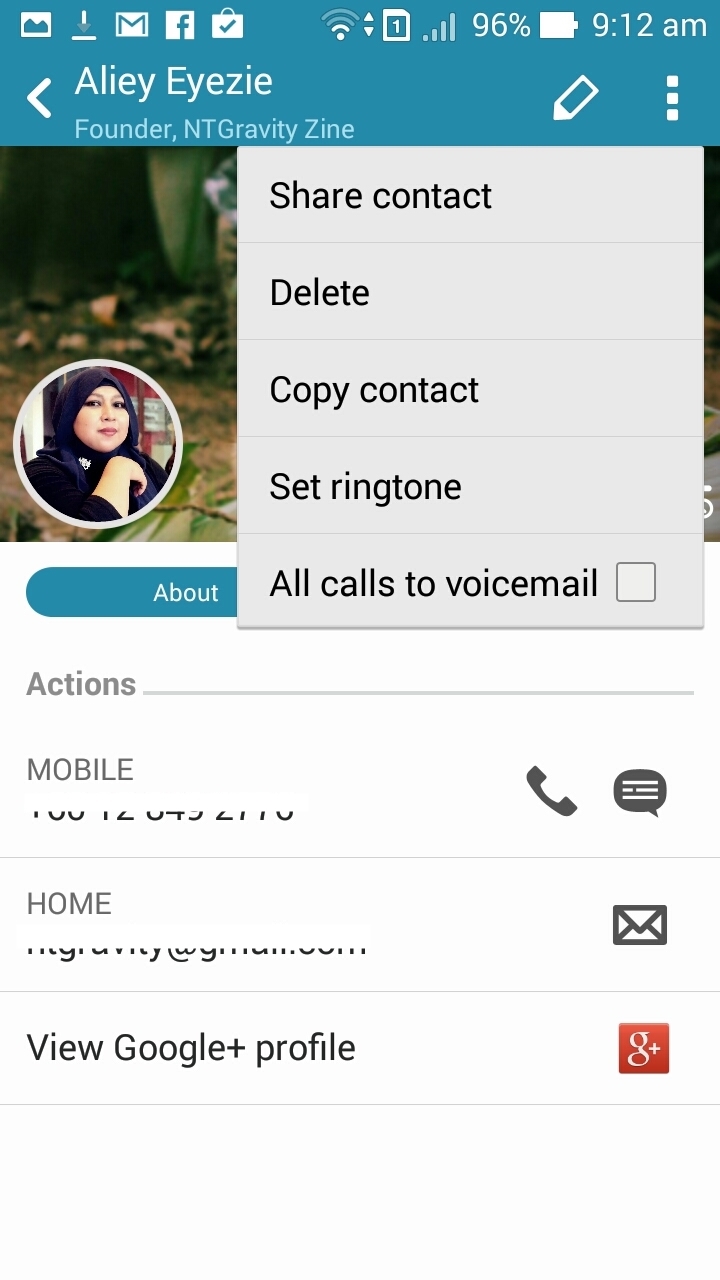This screenshot from a mobile phone contacts app features a sleek blue header with the contact's name, Ailey Eisey, prominently displayed. Ailey Eisey is noted as the founder of NTGravity Zine. The dropdown menu is expanded, revealing options such as "Share Contact," "Delete," "Copy Contact," "Set Ringtone," and "All Calls to Voicemail."

Below the header, Ailey's profile picture is visible inside a circular frame. She is wearing a head covering and a black shirt. Directly under the photo, there is a blue "About" button. The contact details include sections labeled "Actions" and "Mobile," accompanied by a phone icon and a talk button.

Additional information includes a "Home" line featuring an email icon and a link to view her Google+ profile. The Google+ icon is clearly visible as a red square with a "G+" symbol in white. This comprehensive screenshot offers a detailed view of Ailey Eisey's contact page on a mobile device.